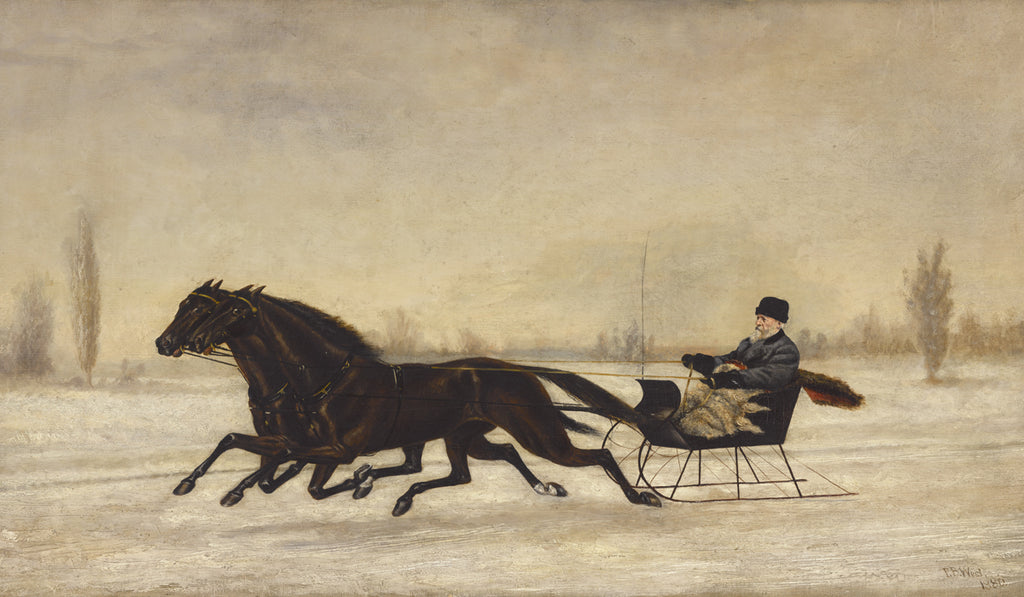This colored artwork, possibly an old print or painting, depicts a dramatic winter scene set against a snowy and muted cream landscape under a cloudy sky with patches of gray. In the foreground, a black sleigh with curled blades glides swiftly from the right to the left, pulled by two dark brown, nearly black, horses adorned with head accessories, galloping at full speed. The elderly white man sitting on the sleigh is wrapped in a white and gray blanket, wearing a heavy gray coat, black gloves, and a black hat. His white beard and mustache are visible, and a scarf billows behind him, adding to the sense of motion. Sparse trees and bushes, devoid of leaves, dot the background, emphasizing the cold and desolate winter setting. The smooth, untouched snow on the ground suggests that the man and his horses are the first to traverse this landscape.